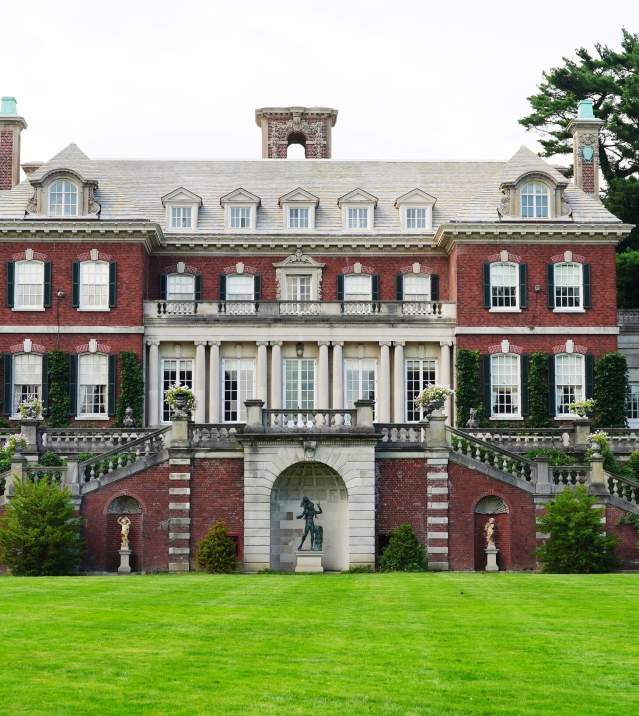The photograph showcases a grand, three-story Victorian-style mansion set against a clear sky. In the immediate foreground, an immaculately cut, bright green lawn stretches out, adding a touch of pristine elegance to the scene. The mansion, constructed of brick-red and accented with darker hues, features an array of long windows framed by classic columns. Centered at the front of the building is an alcove housing an enigmatic statue, flanked by staircases descending on either side. On the roof, dormer windows and a prominent chimney are visible, while several meticulously maintained bushes are strategically placed around the area, enhancing the overall sophisticated ambiance. The serene setting and architectural details evoke a timeless, refined aesthetic, making it a quintessential image of opulence and classic charm.